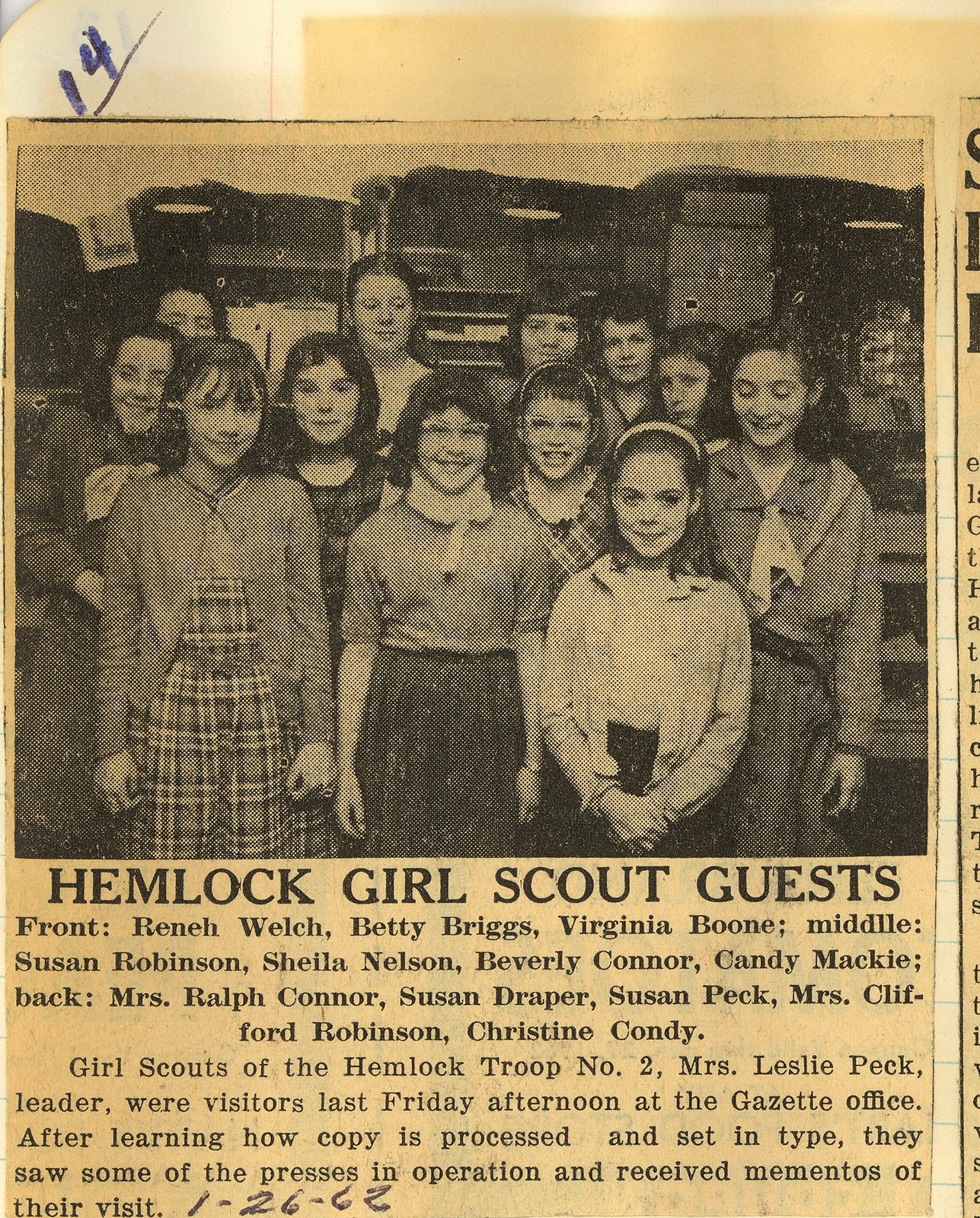This image is a rectangular-shaped, old newspaper clipping, yellowed with age, and printed on almost light tan paper, though parts of it still retain some white. On the upper left-hand corner, someone has written the number "14" diagonally in blue ink. Taking up about two-thirds of the clipping is a black-and-white photograph depicting approximately twelve young, Caucasian girls, some in Girl Scout uniforms, standing in three rows. Below the photograph, in bold black print, is the title "Hemlock Girl Scout Guests." 

The names listed under the photograph specify the girls' positions: 

- Front row: Renee Welch, Betty Briggs, Virginia Boone
- Middle row: Susan Robinson, Sheila Nelson, Beverly Conner, Candy Mackey
- Back row: Mrs. Ralph Conner, Susan Draper, Susan Peck, Mrs. Clifford Robinson, and Christine Condi.

A paragraph beneath the title provides further details: "Girl Scouts of the Hemlock Troop Number Two, Mrs. Leslie Peck, leader, were visitors last Friday afternoon at the Gazette office. After learning how copies are processed and setting type, they saw some presses in operation and received mementos of their visit." 

Adjacent to this paragraph, handwritten in black ink, is the date 1-26-62.